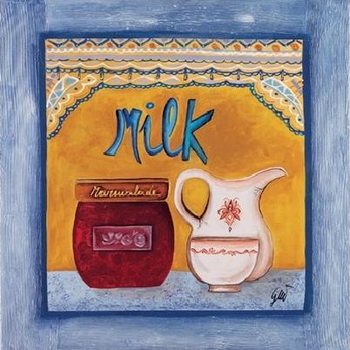The image is a detailed drawing with a primarily blue color scheme, featuring a variety of items arranged on a blue tabletop against an orange backdrop. On the right side of the drawing is a white jug adorned with a floral pattern, placed with its opening facing right and the handle oriented left. In front of the jug is a small white cup edged with a pink border. To the left of the jug, there's a red jar with a wooden-engraved lid, marked as a marmalade jar. Above the jug and jar, the word "MILK" is written in blue, giving a handcrafted feel. Above this text, a blue-yellow patterned curtain is elegantly depicted, adding a decorative touch to the composition. The entire scene is encased in a wooden frame with a brownish-white hue. This aesthetic piece brings together elements of rustic charm and vibrant color.